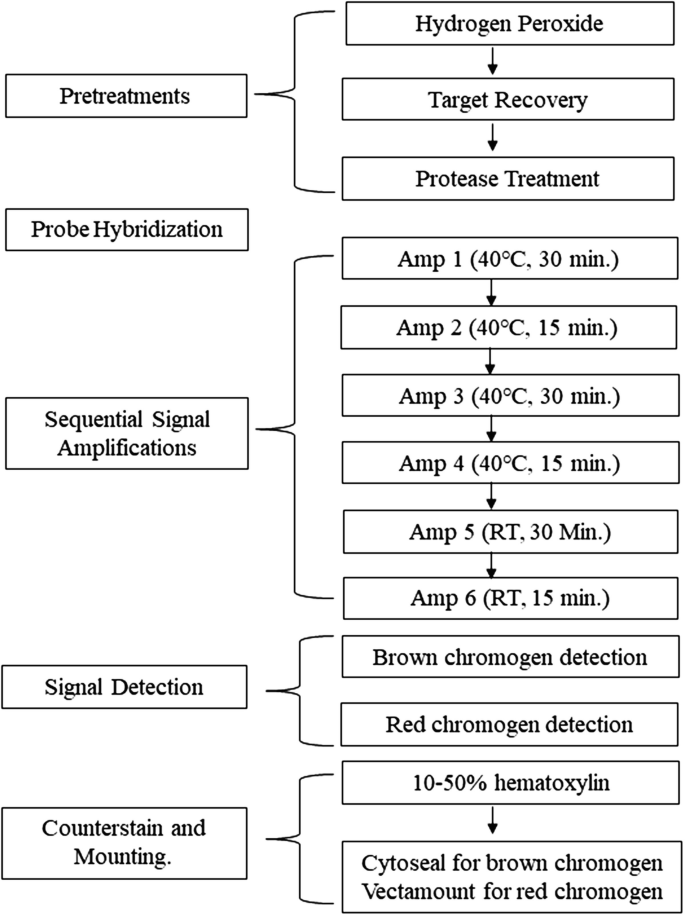This portrait-oriented image depicts a detailed scientific flowchart with a white background, structured with two rows of rectangular boxes featuring thin black borders and captions. On the left, various stages of a process are listed, each connected by small lines and brackets to corresponding steps on the right. 

Beginning at the top, the first leftmost box is labeled "Pre-treatments," branching to the right to three boxes: "Hydrogen Peroxide," "Target Recovery," and "Protease Treatment," each connected by downward arrows. Below is "Probe Hybridization," which has no additional boxes branching off to the right. Following this is "Sequential Signal Amplifications," connecting to six right-hand boxes: "Amp 1, 40°C, 30 min," "Amp 2, 40°C, 15 min," "Amp 3, 40°C, 30 min," "Amp 4, 40°C, 15 min," "Amp 5, RT, 30 min," and "Amp 6, RT, 15 min." 

Next is "Signal Detection," branching out to two boxes: "Brown Chromogen Detection" and "Red Chromogen Detection." Lastly, the flowchart ends with "Counterstain and Mounting," which connects to "10 to 50% Hematoxylin and Cytoseal for Brown Chromogen" and "Vectamount for Red Chromogen."

The chart methodically outlines a scientific process, transitioning from pretreatments to detailed signal amplifications, and concluding with signal detection and sample stabilization through counterstain and mounting.